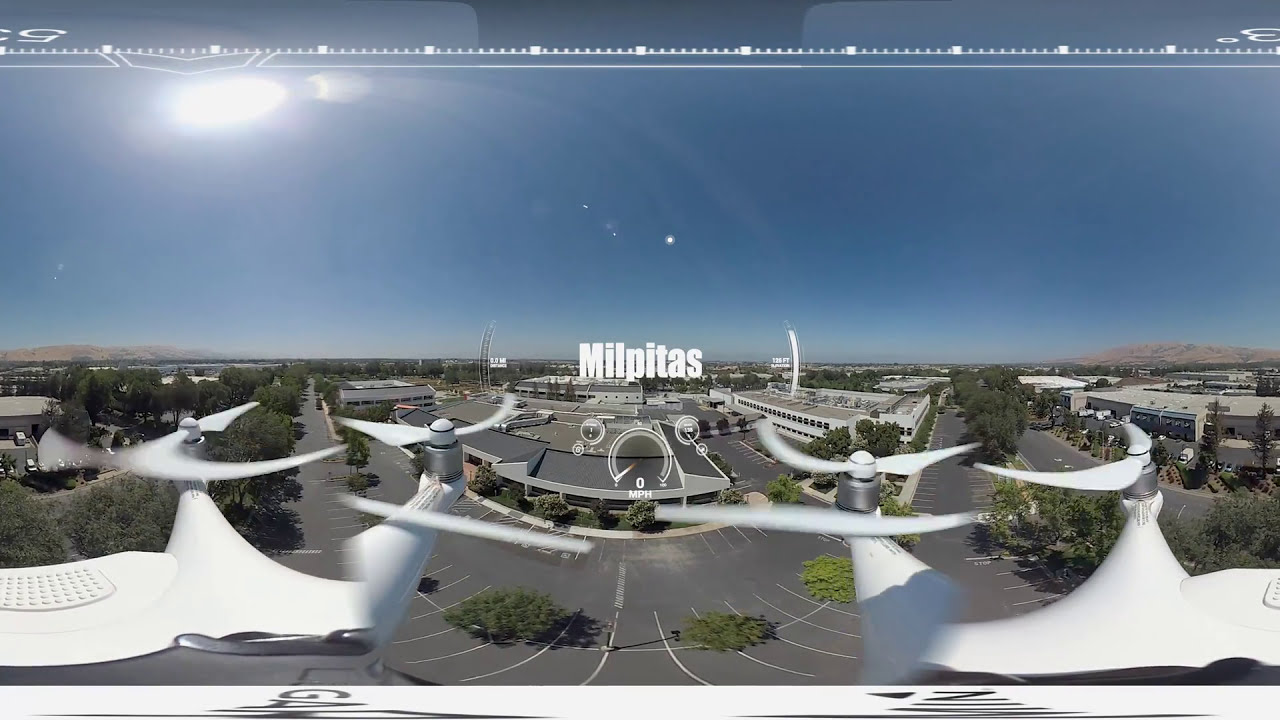The panoramic image, captured from above by a drone or an eVTOL (electric Vertical Take-Off and Landing) aircraft, prominently features a striking interplay of colors and elements. Dominated by white, the photograph showcases a landscape that melds structure and natural beauty. In the foreground, several multi-rotors suggest the presence of cutting-edge aerial technology, possibly helicopters or drone propellers, indicating a scene of dynamic movement. Below these propellers, roads interspersed with green medians snake through the area, leading towards a central rounded building that seemingly serves as an office space.

Amid this intricate composition, there's a distinct sign centered in the background reading "Milpitas," hinting at the image’s Californian locale. This sign is flanked by references to the drone’s data, such as coordinates and speed displays, contributing to the high-tech vibe of the scene. Enhancing the depth of the image, a vibrant blue sky stretches across the top, while tree-dotted roads lead the eye towards distant mountains on both sides. The sun blazes high in the sky, casting a bright, clear light over the putative transportation center below. The overall scene is bustling yet harmonious, capturing a blend of modern transportation against a serene natural backdrop.